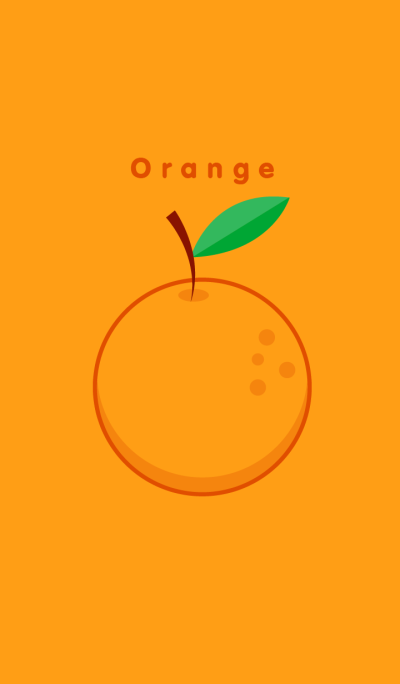The image features a vertically oriented, simplistic illustration centered around the theme of the color orange. The background is a light orange hue, setting the stage for a sketched depiction of an orange fruit prominently placed in the middle. The fruit itself is outlined in a darker shade of orange, with medium orange spots and shadows adding depth. A brown stem and green leaf—light green on top fading into a darker green on the bottom—adorn the fruit. Above the orange, the word "orange" is inscribed in dark orange text, with an uppercase "O" followed by lowercase letters. This minimalistic yet effective design uses a cohesive color palette predominantly of oranges, greens, and browns, creating an appealing and educational visual that could easily be used in a classroom setting to teach young children about colors, shapes, and fruits.